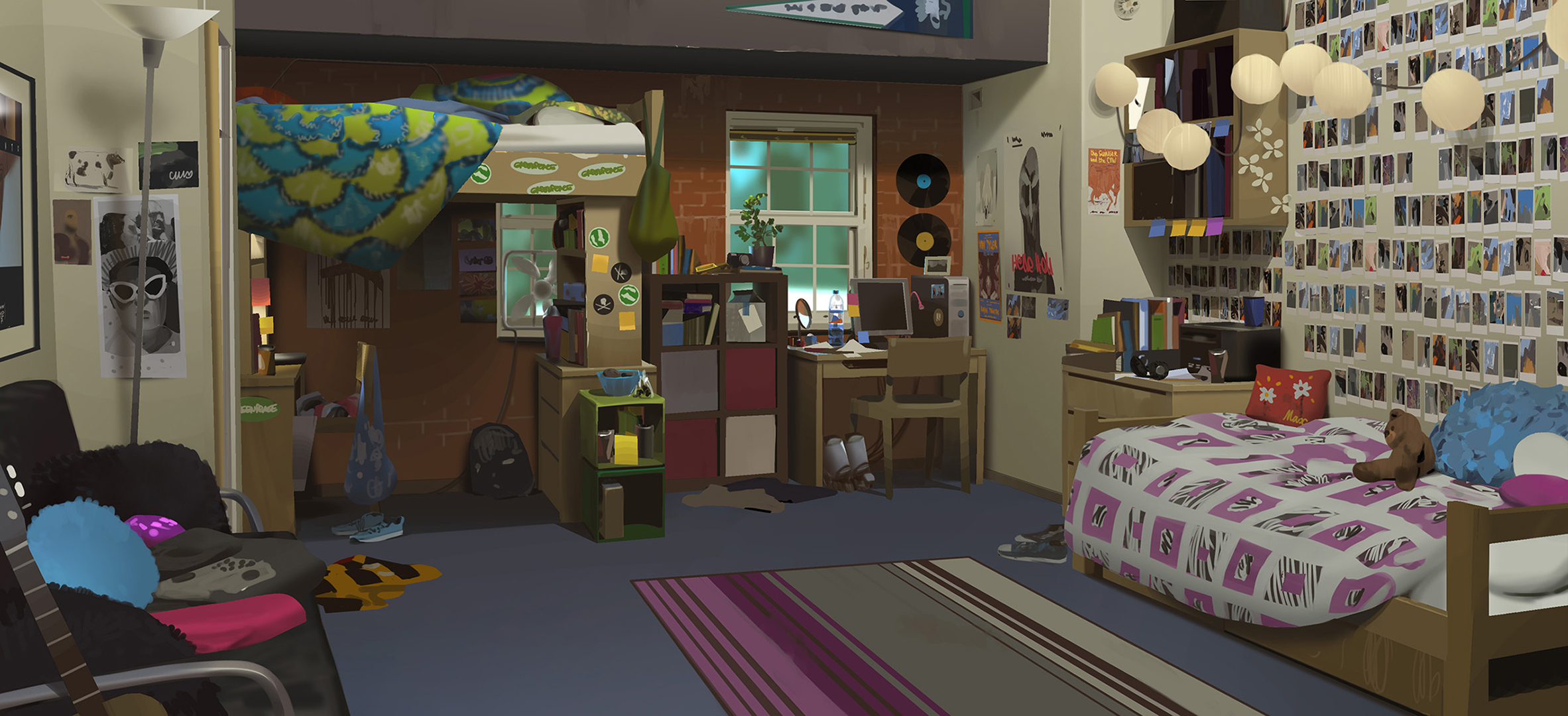This image depicts a digitally rendered, realistic bedroom, likely created using a program like The Sims or Photoshop. The room features a bed adorned with a white and purple covering and a teddy bear, positioned against a white-painted brick wall. On the wall above the bed, there are numerous Polaroid pictures, colorful decals, records, and posters meticulously arranged. The floor boasts both a blue rug and a pink, gray, and white area rug. Furnishings include a tan desk with a computer, a white floor lamp, a guitar, and a chair. Notably, there is a bunk bed setup with no visible ladder, raising questions about accessibility. The bottom part of the bunk bed comprises two dressers and a futon. Scattered around the floor are a pair of sneakers and a backpack. The room also has two windows; one features a fan. Overall, the detailed placement and varied elements contribute to a cluttered, dorm-like atmosphere, highlighting the room's blend of homely and chaotic vibes.